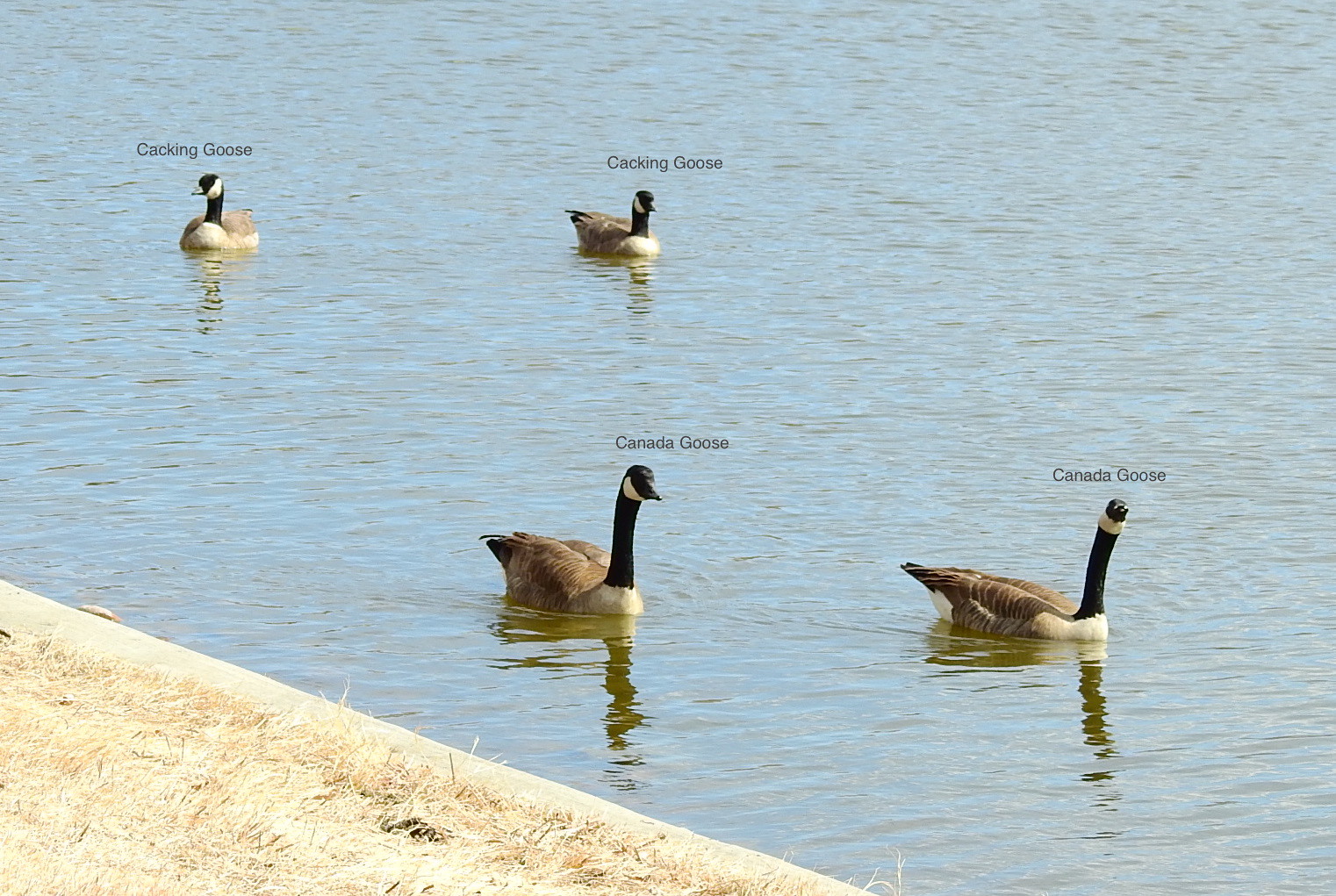The image is an outdoor, color photograph featuring a tranquil scene on a wide body of water with a light blue hue, accented by grayish ripples and reflections. Four geese are seen swimming in the water, each identified by black text labels above their heads. The two geese in the upper part of the image are labeled "Cackling Goose," while the two geese in the lower part are labeled "Canada Goose." These birds have distinctive black necks and beaks, white markings under their chins, lighter brown feathers on their bodies, and black tail feathers. In the bottom left corner of the image, a concrete barrier and a patch of withered, yellow-brown grass can be seen.